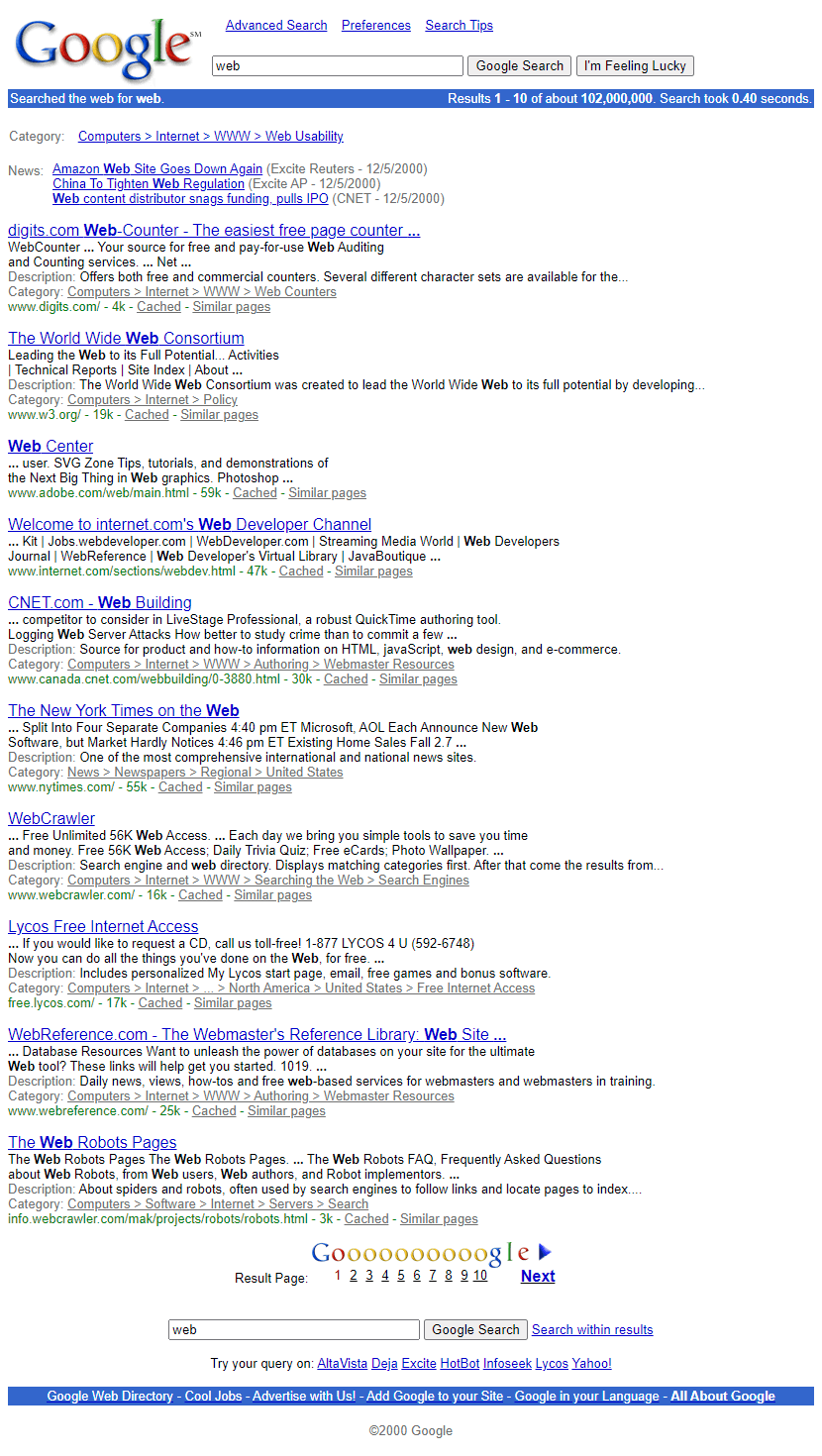A nostalgic glance at an early iteration of the Google search page. The simple, clean interface includes several characteristic blue hyperlinks such as "Advanced Search" and "Preferences." Prominently displayed at the center is the quintessential Google search bar, accompanied by the iconic "Google Search" and "I'm Feeling Lucky" buttons. Below the search bar is a list of search results featuring phrases like "web counter," "worldwide web," and "welcome to internet.com," offering a glimpse into the early internet landscape and its seminal web services like CNET and WebCrawler. A large blue bar divides sections of the page, symbolizing the straightforward and utilitarian design ethos of early web interfaces. The unmistakable logo and numerical pagination (1 through 10) to navigate multiple search results pages are hallmarks of the Google's initial approach to organizing the vast expanse of the web.